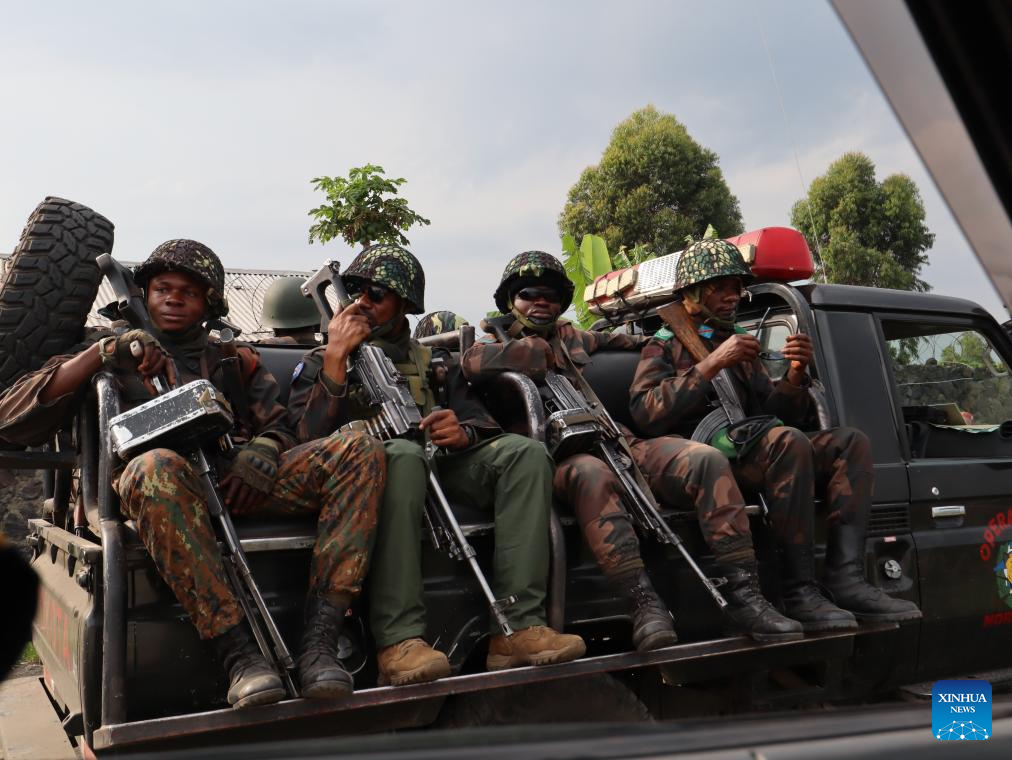The image depicts an outdoor scene during the day, capturing a military pickup truck in a dark army green color with a red flashing light on the roof, which could indicate it's a medical or command vehicle. In the back of the truck, there are seats occupied by at least four soldiers on the visible side, all facing towards the camera. The soldiers are wearing full military gear, including camo uniforms, helmets, black army boots, and sunglasses. Each soldier is holding a large automatic weapon, identifiable by their prominent metal parts. Specifically, the visible soldiers include three Afro-American men and one who appears to be Caucasian or Afro-American, all with similar camouflage attire and rifles. In the background, trees can be seen, providing a natural setting. Notably, the bottom right corner of the image is marked with "Xinhua News," indicating the photo's possible origin or credit. The truck also has a spare tire mounted on the back.